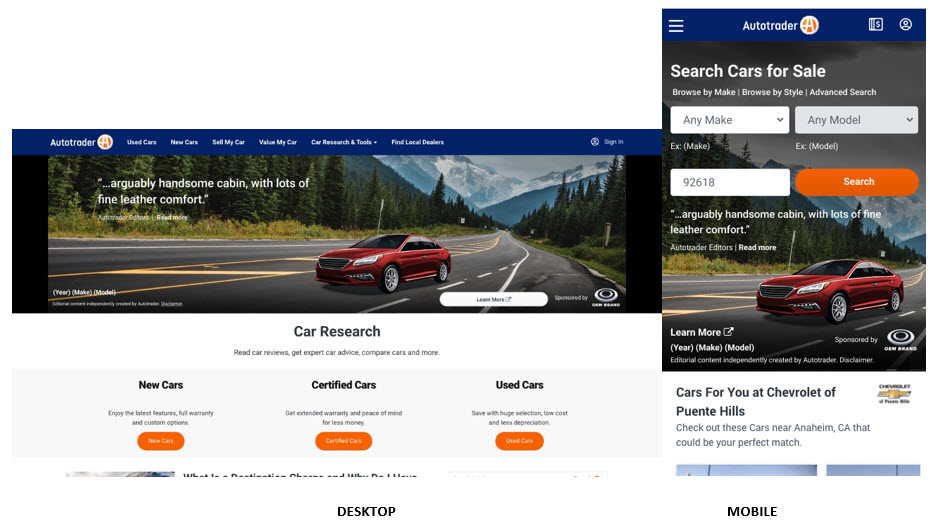The image captures a webpage from AutoTrader. On the left, the AutoTrader logo, a white circle with an orange center and a white 'A', is prominently displayed. The main navigation bar features several tabs in a dark blue bezel, including "Used Cars", "New Cars", "Sell My Car", "Value My Car", "Car Research & Tools" (with a dropdown menu), and "Find Local Dealers". 

Central to the webpage is an image of a red car seemingly superimposed on a roadway. The road is dark gray with a central yellow lane, commonly known as a "suicide lane", and is flanked by dark green trees. The background showcases mountains; some have snow-capped peaks appearing blue in the distance, while others are greener. There are additional green and yellow hues on either side of the road. Below the car image, a bold black headline says "Car Research". Regular black text beneath it provides information on reading car reviews, getting expert advice, comparing cars, and more.

The section about new, certified, and used cars follows. In a light gray rectangle, the bold black header "New Cars" is accompanied by text explaining the benefits of new cars, such as the latest features, full warranties, and custom options. A clickable dark orange oval button with white text invites users to explore new cars further. The "Certified Cars" section highlights obtaining extended warranties and peace of mind for less money, with a similar dark orange button labeled "Certified Cars". The "Used Cars" section emphasizes savings through a large selection of low-cost vehicles with less depreciation, providing a button for used car listings.

At the bottom, categories such as "Desktop" and "Mobile" are in bold, indicating different site views. The mobile version features three white lines in a dark blue bezel and centers the AutoTrader logo. Below, there is a dark blue square with a dollar sign and a white circle with a person's silhouette. The black background image includes blue mountains with white caps, repeated imagery of the red car, and bold white text "Search Cars for Sale". Below, options for browsing by make and style, as well as "Advanced Search", are available. Drop-down rectangles for "Any Make" and "Any Model", an "Ex(Make)" field, an "Ex(Model)" field, a white rectangle with "92618", and an orange search button with white text facilitate searches. A quotation with ellipses reads: "Arguably handsome cabin, with lots of fine leather comfort," credited to AutoTrader editors. A hyperlink in bold white text, "Read More," is available for further details. At the very bottom, the text "Cars for you at Chevrolet of Peanteehills." concludes the webpage.

This comprehensive caption encapsulates all elements and textual information present on the AutoTrader webpage, providing a thorough, detailed overview.